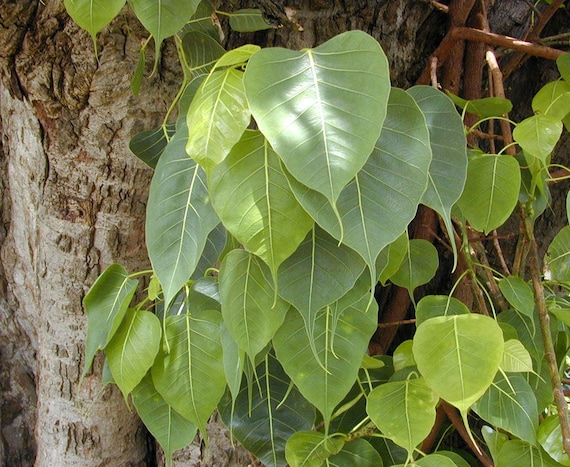In the image, a large, aged tree trunk with dark, rough, and deteriorating bark dominates the scene. The bark, peeling in places, exhibits multiple shades of brown and has a highly textured surface with pointy sections. Climbing up the side of this ancient tree are large, frond-like ivy leaves featuring a prominent central vein with horizontal lines extending outwards. These leaves vary in size and display a spectrum of greens—ranging from dark green to pale yellow-green. The variation in color seems to depend on the amount of sunlight each leaf receives, as most leaves remain in the shade with only one reflecting bright sunlight. Additionally, there are clusters of dark and light brown twigs and branches, seemingly old and intertwined, accompanying the leaves. Some of these leaves have their own support stems but are using the tree to maintain their structure and balance.